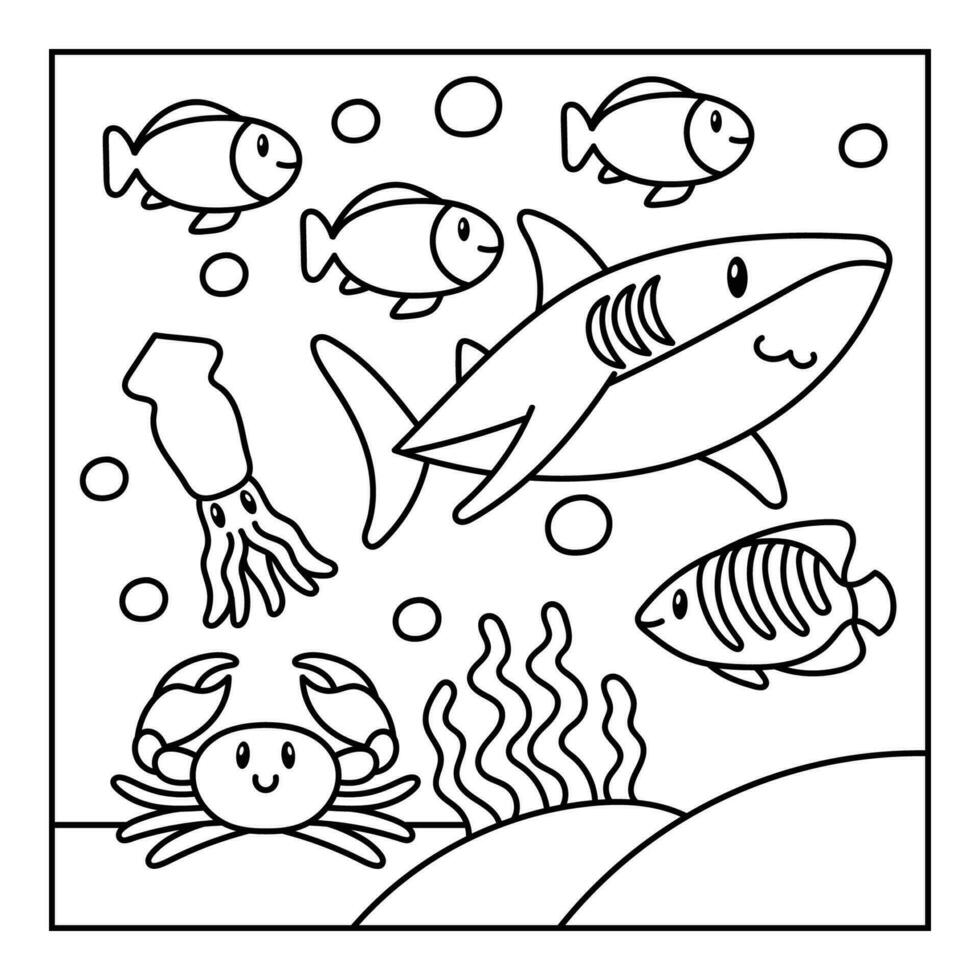This is a simple black-and-white line drawing, reminiscent of a kid's coloring book, depicting an underwater scene in a cartoony style. Central to the illustration is a shark with a smirk, drawn in the middle right portion of the image, facing to the right. To the left of the shark is a squid, and below it, a smiling crab with tentacle-like legs stands on a flat area of the seafloor. To the right of the crab, there is a striped fish facing left, positioned on the bottom right of the image. At the top of the drawing, three identical small fish with rounded faces swim horizontally to the right, with the middle one slightly lower. Various bubbles are scattered throughout, including eight distinct air bubbles rising between the sea creatures. The seafloor features rolling hills, created with simple arcs, and some squiggly lines depicting underwater plants at the very bottom center.